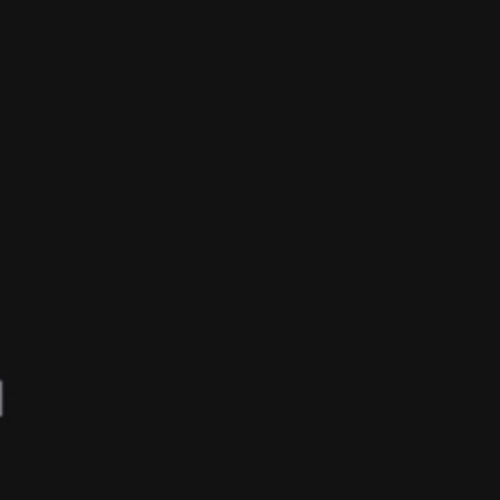A minimalist image featuring a large, solid black square centered against a plain white background. The black square is uniform in size on all sides, with no visible text, images, or patterns within or around it. The simplicity of the square against the stark white backdrop suggests no additional context, elements, or information, providing a purely abstract composition. The origin of the image—whether from a computer or a phone app—is indiscernible, emphasizing its fundamental and unembellished nature.